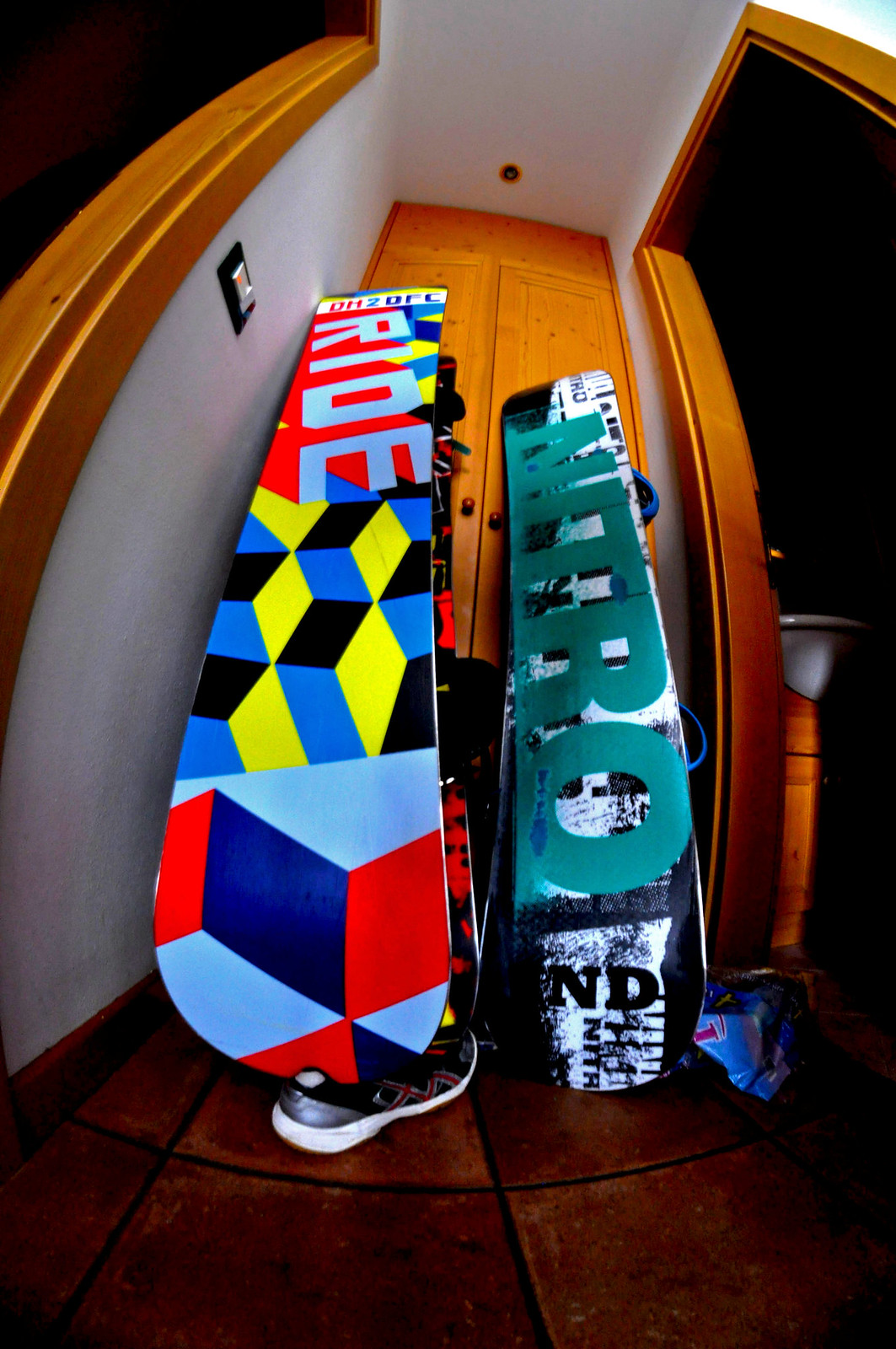This photograph, taken from a low angle near the floor, reveals a partial view of a hallway in a house, with a brown cabinet extending from the floor to the ceiling on the left side of the image. Resting against the cabinet are two snowboards. The snowboard on the left is vibrant and multicolored, featuring geometric patterns in shades of black, blue, yellow, and red. At the top, orange text reads "RIDE" with additional smaller text "DH2DFC" in various shades of red and blue. The snowboard on the right showcases a more monochromatic design with black, white, and teal colors, prominently displaying the word "NITRO" in green capital letters and "ND" in smaller black letters at the bottom. A black and red shoe can be seen under the snowboard on the right, and the scene is set on a brown-orange tiled floor beneath a white ceiling.